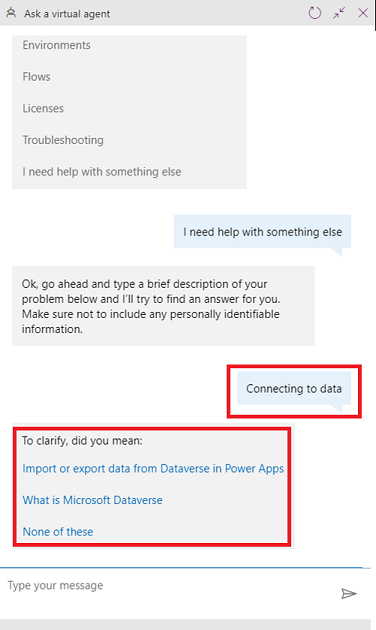The image displays a user interface featuring a detailed chatbot interaction. At the top of the screen is a light gray banner with the text "Ask a Virtual Agent" accompanied by a robot icon. Adjacent to this on the opposite side is a purple semi-circle with a double-arrow icon.

Below the banner, on a white background, is a lighter gray square containing multiple categories in capital letters: "Environments," "Flows," "Licenses," "Troubleshooting," and "I Need Help with Something Else." The category "I Need Help with Something Else" is displayed in black text within a light blue response box.

Following the user’s selection, a dialog box appears with instructions: "Okay, go ahead and type a brief description of your problem below and I'll try to answer for you. Make sure not to include any personally identifiable information." The system begins connecting, indicated by a red-bordered message that says, "Connecting to data..."

Another red-bordered dialog box appears with the prompt, "To clarify, did you mean," followed by several blue text options: "Import or export data from Dataverse in Power Apps," "What is Microsoft Dataverse," and "None of these." At the bottom, a blue line indicates where the user can type their message.